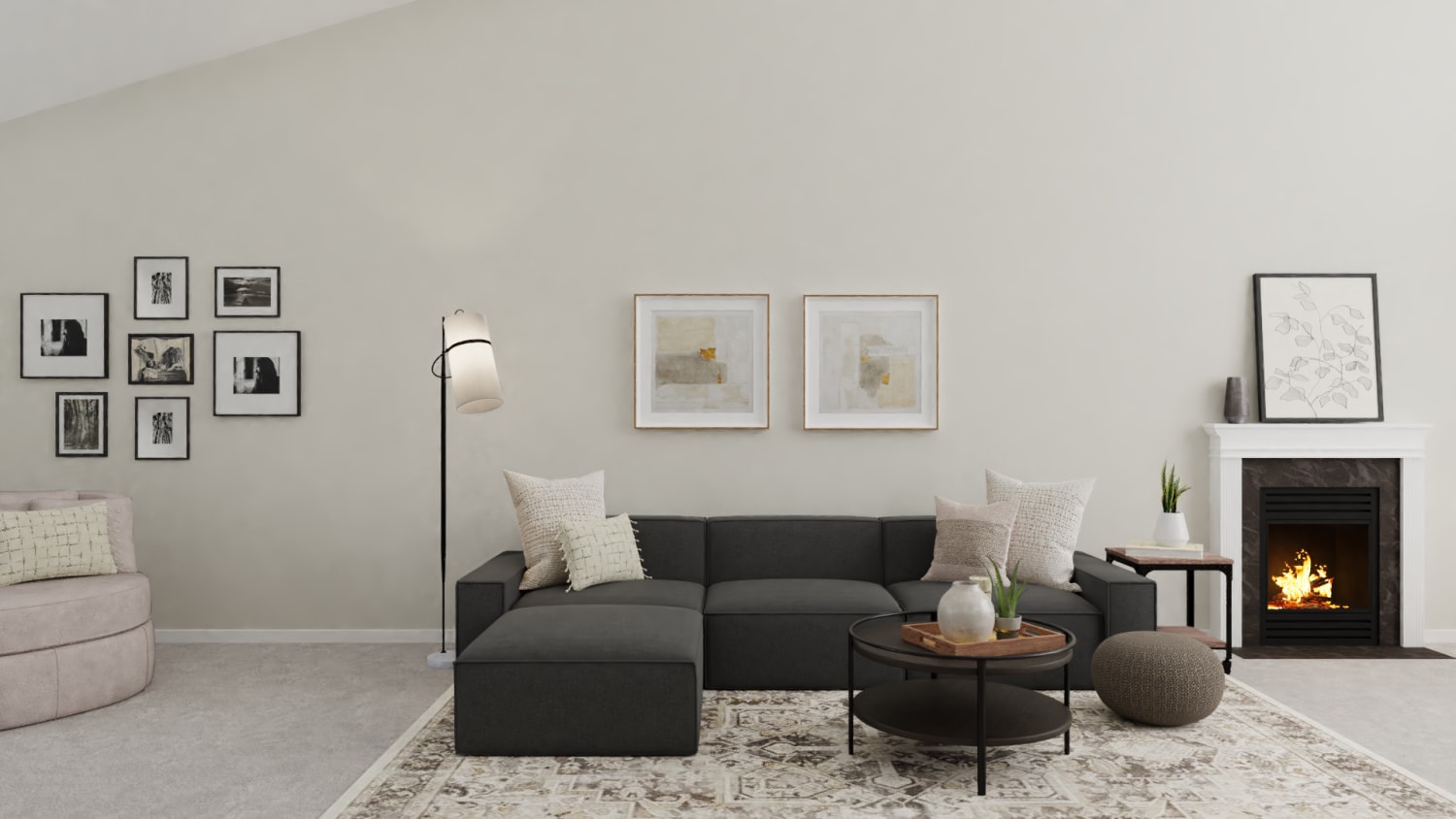This image depicts a cozy living room featuring predominantly eggshell-colored walls. On the left side, there is a distinctive arrangement of black-framed, black-and-white photos organized in a circular pattern around a central picture. Forward of this gallery is a white or off-white round chair. Centrally located in the room are two muted pastel, abstract pictures in gold frames with white mattes. Beneath these artworks lies a gray sectional couch, which includes a lounge chaise and is adorned with two white pillows. In front of the couch, a small, round black coffee table is positioned on an abstract white and gray rug. The coffee table holds a tray with a small ceramic pot and a plant. To the couch's left, there's a white lamp and a side table, while the right side of the couch features a small corner stand. A little brown poof provides extra seating or a place to rest your legs. Additionally, the right side of the room showcases a fireplace adorned with a drawing, further contributing to the room's inviting atmosphere.